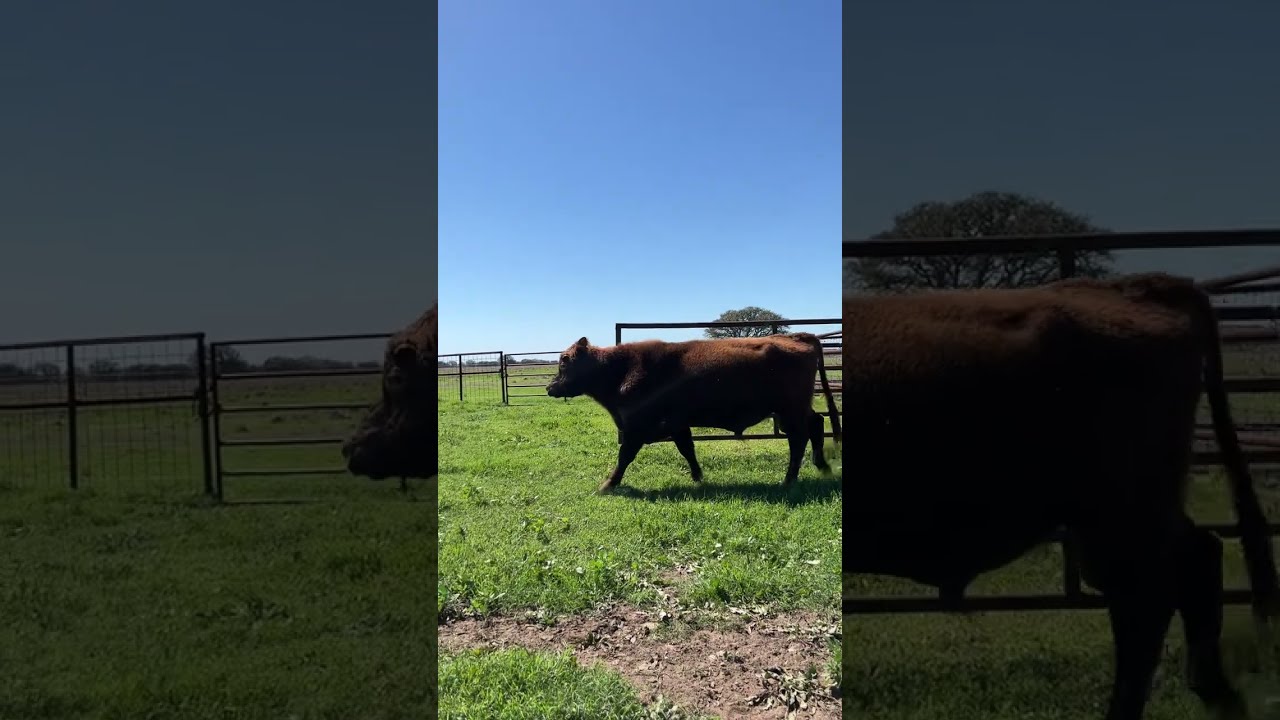In a vivid outdoor daytime setting on a farm, the image captures a large, pure brown cow walking to the left on a verdant grassy field. The still shot, seemingly a phone picture displayed within a video frame, shows the cow's body highlighted in the center with brighter colors, while the edges fall into shadow. The horizontal rectangle image is sectioned, with a vertical inset emphasizing the cow. Behind this central figure, a metal fence and gate are visible, with a blue, cloudless sky arching above. A tree stands in the distance, and the ground right in front of the cow shows a patch of bare, light gray dirt amidst the abundant green grass. The serene scene is devoid of text, focusing solely on the natural farm environment.